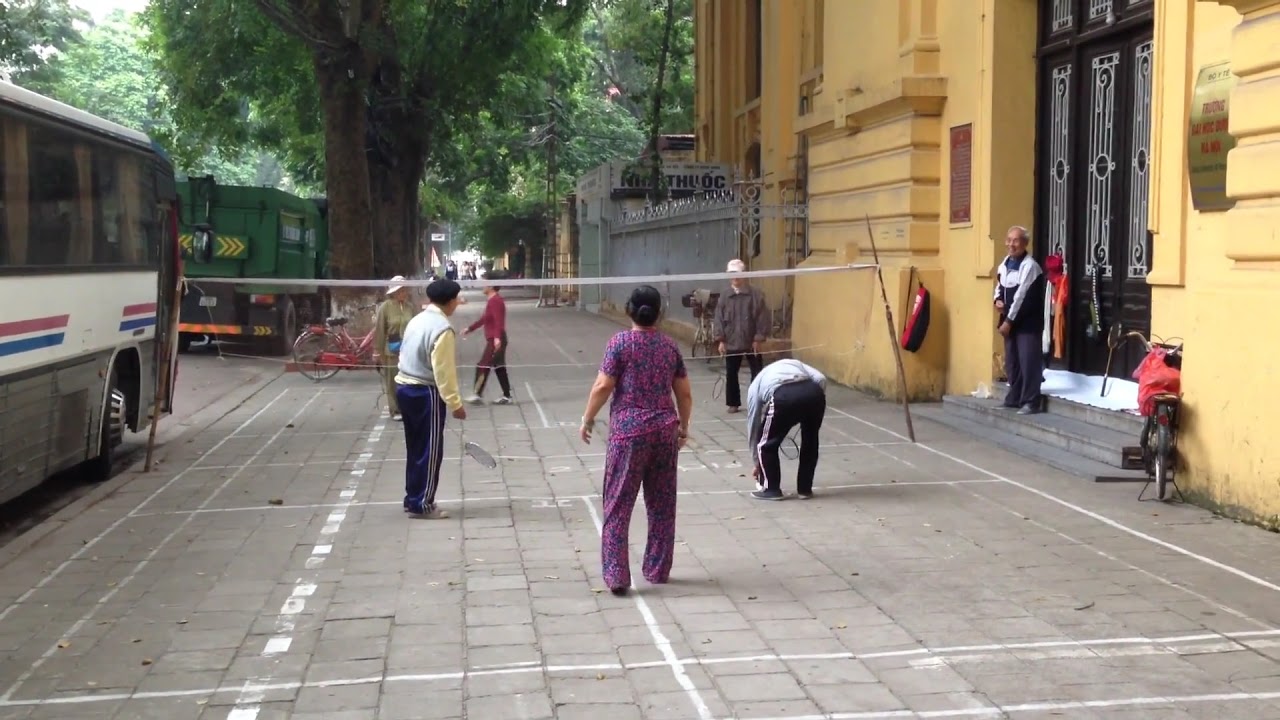On a wide, stone-tiled public sidewalk outlined with white chalk for a badminton court, various older individuals enthusiastically engage in a game of badminton. A white and black net, held up by two wooden poles, stands in the center, with players holding rackets positioned on either side. A tall yellow building with black doors and white-paned windows overlooks the scene on the left, and a black bicycle with a vibrant red jacket is propped against one of the doors. To the right, a blue and white bus with red and blue stripes, and a green garbage truck, are parked by the street, adding to the urban backdrop of this lively and cheerful outdoor activity.